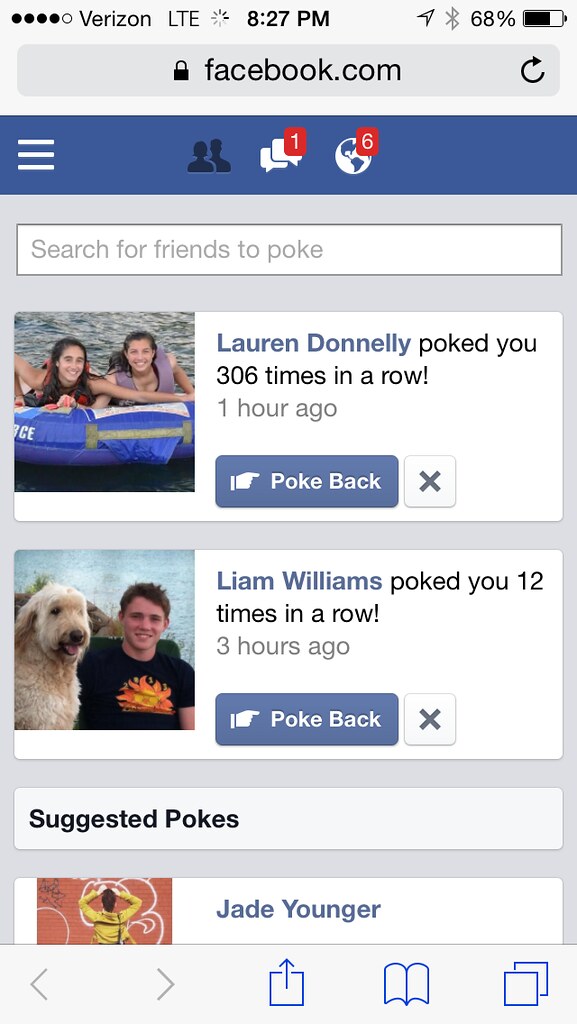This image is a vertical, rectangular screenshot of a Facebook page viewed on a Verizon LTE phone with a battery charge of 68%, taken at 8:27 PM. The top status bar includes the Verizon LTE label, time, and battery percentage. Below this, the grey navigation bar displays "Facebook.com," and under it, there's a blue bar featuring profile icons with a red notification badge displaying the number "1" and a globe icon with "6" alerts. The search prompt reads "Search for friends to poke."

Highlighted prominently are two notifications: one from Lauren Donnelly, who poked the user 306 times an hour ago, and another from Liam Williams, who poked the user 12 times three hours ago. Both entries include a "poke back" option. Lauren Donnelly's profile picture shows her and another young girl on a plastic raft in what appears to be a river, while Liam Williams' image features him in a black t-shirt next to a dog outdoors. The page is organized to track poke notifications and includes a suggested poke section beneath the main notifications.